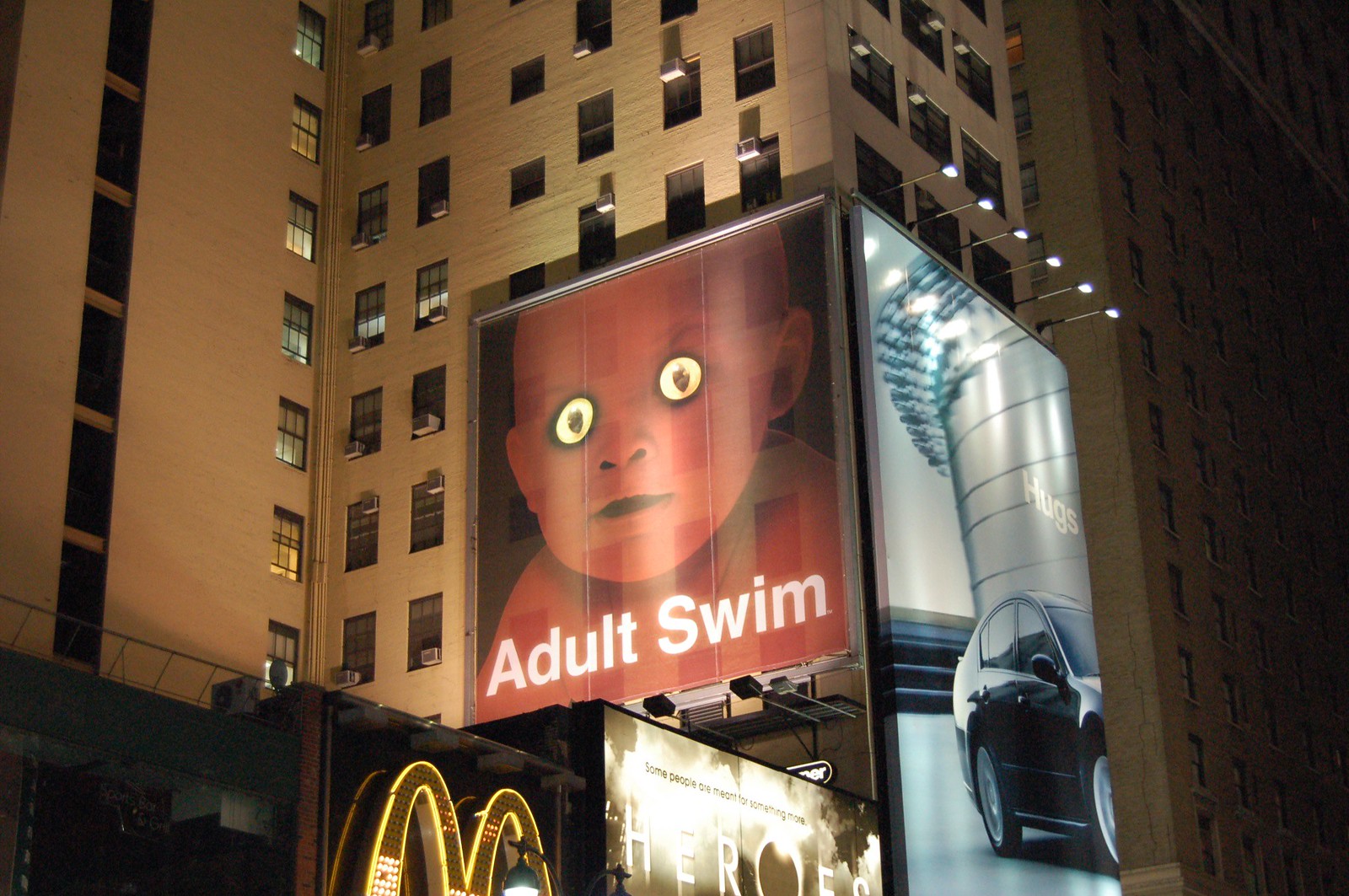This image captures a nighttime scene in New York City, showcasing the side of a very tall building, potentially an office or apartment complex, adorned with multiple windows, some equipped with window-style air conditioners. The focal point is a series of billboards: prominently, there is an eerie red baby with wide-open, glowing yellow eyes and strange pupils, promoting Adult Swim in white letters below. Adjacent to it, on one side, there's an advertisement for a car with the word "hugs" visible. Below, the McDonald's golden arches are illuminated, and another billboard advertises the show "Heroes." This snapshot, likely taken around 2007 or 2008, captures the bustling, illuminated essence of an iconic urban landscape.